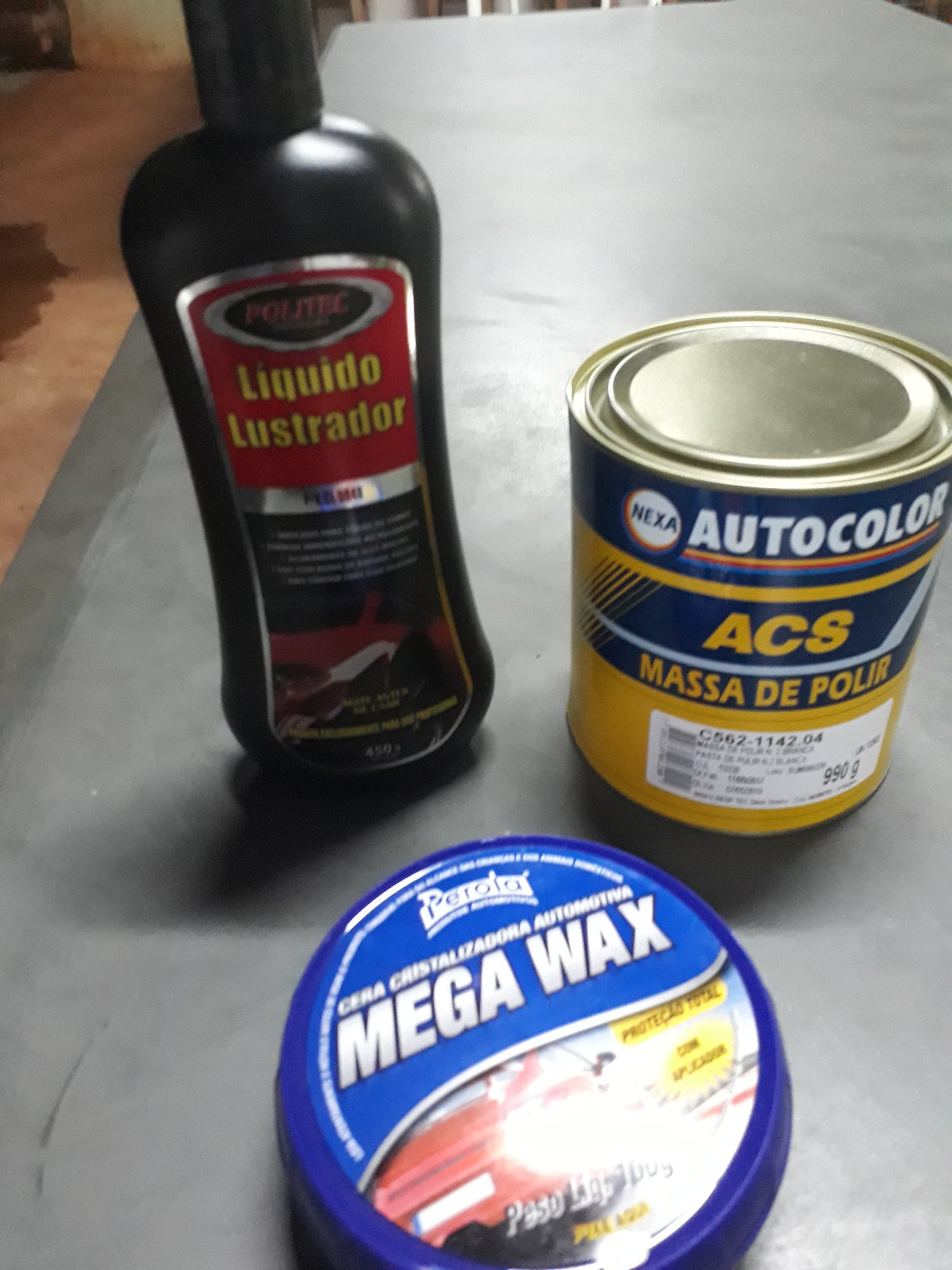This image depicts a close-up of three automotive products arranged on a gray table, likely situated in a shop environment, given the visible floor with what appear to be oil or water stains. To the left, there’s a tall, dark brown bottle labeled “Líquido Lustrador” with a cap on it and a car image at the bottom, hinting at its use for auto detailing. The label is a mix of red, black, and silver colors. In the center of the photo, there is a blue cylindrical can of “Megawax,” featuring a red car on its label, suggesting it is a car wax protectant. The product name is written in white lettering. To the right side, there's another can colored blue and yellow, with the wording “Nexa Autocolor ACS Masa De Polar” prominently displayed. This can also has a white label with a barcode and other numbers. The yellow and white text stands out against the blue background, indicating it might be an auto paint-related product. The careful arrangement of these items on the stand highlights their purpose in automotive care and maintenance.